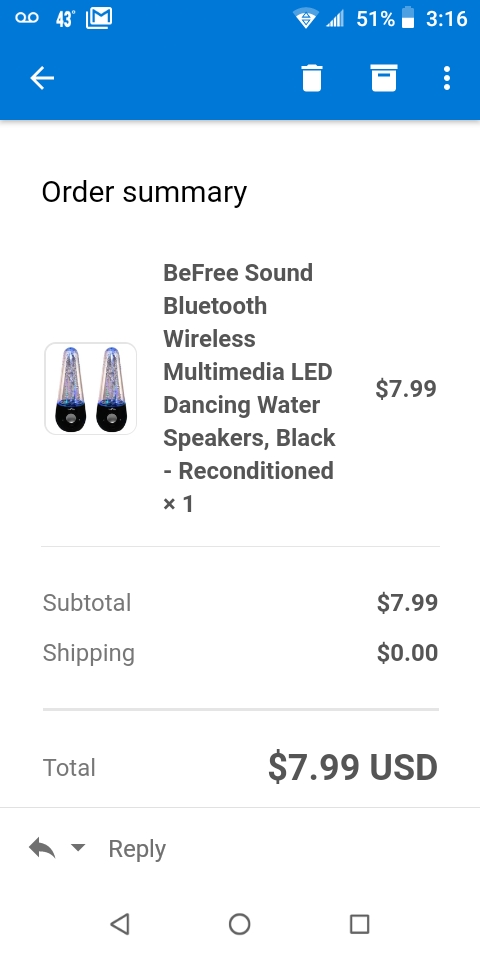This image showcases an order summary for a product. The order details are structured from top to bottom on the screen. The ambient temperature is displayed as 43 degrees, and the phone's battery is at 51%. A timestamp shows the time as 3:16. Icons for trash and another unspecified function appear on the screen.

The main section of the image presents the order summary. An image of the product is positioned on the left, while the product description and pricing are in the center and right respectively. The product ordered is a BeFreeSound Bluetooth Wireless Multimedia LED Dancing Water Speakers, black and reconditioned, with a quantity of one. The cost of the speakers is $7.99, with a subtotal matching at $7.99. Shipping is free, thus the total cost is $7.99 USD. Below the total, there is a ‘reply’ button.

The visual representation of the speakers indicates they are primarily black at the base, with possibly silver or gray buttons. The top section features clear and blue materials, seemingly containing water-like substances within the product design.